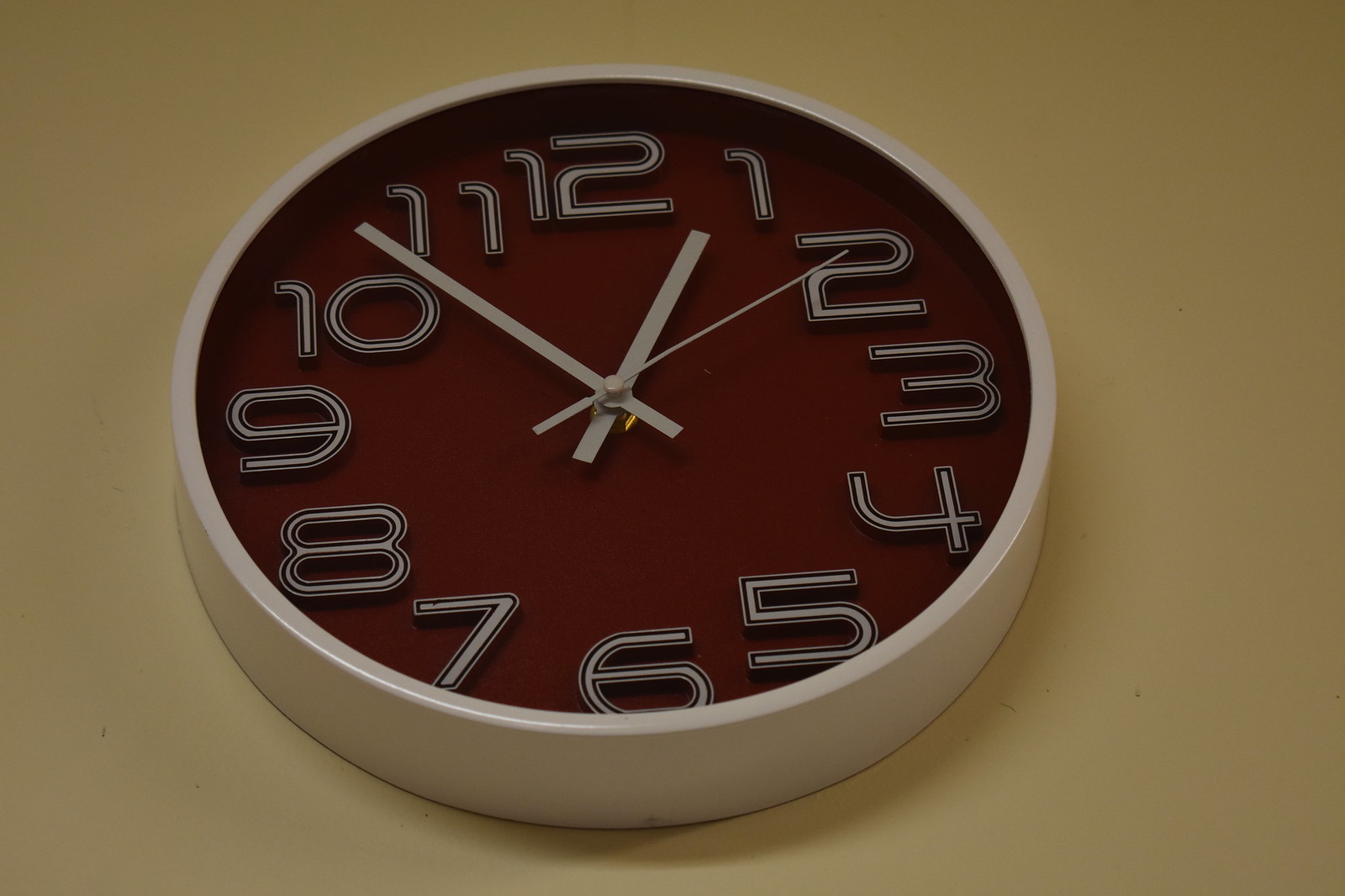This image features a distinctive wall clock with a brown face, deviating from the more common white-faced clocks. The clock displays the numbers 1 through 12 in a gray color with brown borders, enhancing their visibility against the brown background. The gray hour, minute, and second hands are sleek and match the clock's outer gray rim. The time shown is approximately 12:53 and 9 seconds. The clock's background is a light brown painted wall, which complements the clock's unique aesthetic. Notably, there are no brand markings or company names visible on the clock's face.